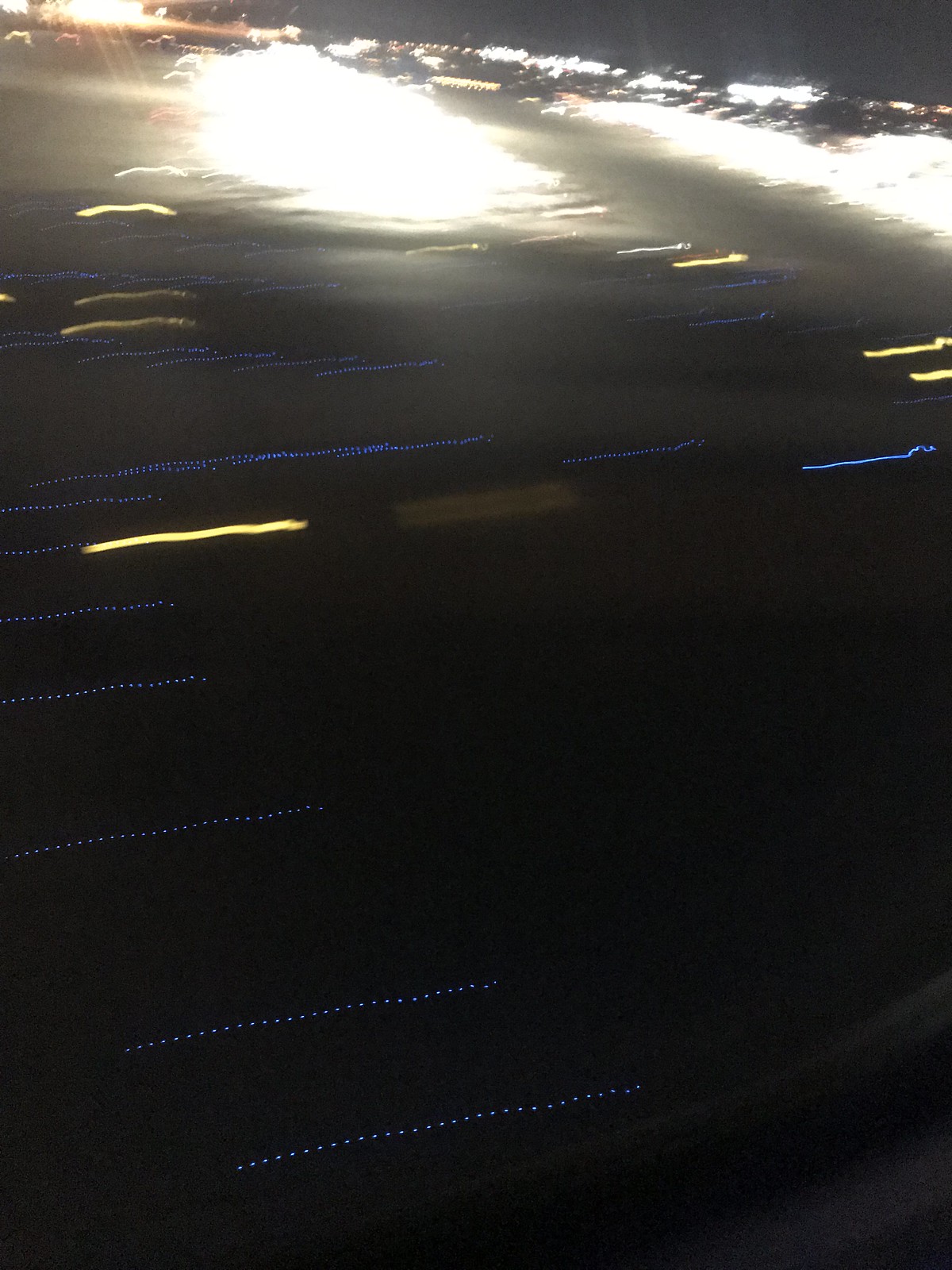In this dynamic, fast-paced photograph, a predominantly dark background is illuminated by a flurry of vibrant light trails. Near the bottom of the image, blue dots speckle the scene, gradually transitioning into elongated yellow streaks as the eye moves upwards. The black background varies in intensity, with patches of gray interspersed throughout. Two significant bursts of light dominate the upper portion of the frame: one centrally placed, the other slightly off to the side. In the hazy backdrop, faint outlines of buildings and cars emerge, suggesting an urban environment. The erratic patterns of light convey a sense of rapid motion, as if captured in a moment of high-speed frenzy or due to a quickly flashing camera shutter. The overall effect paints a lively and chaotic night scene, teeming with energy.